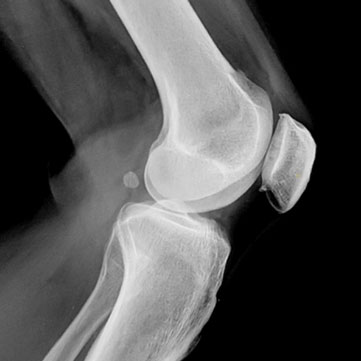The image depicts a black-and-white x-ray, likely of a bone joint that resembles a knee. The top bone is placed diagonally from the center, angling towards the left, while the bottom bone extends diagonally downwards, appearing somewhat tooth-like but elongated, and angles from the top right to the bottom left. At the joint where these two bones meet, a smaller piece of bone can be seen on the top right side. Additionally, there's a small round dot in front of the connection point of the bones, and a rectangular shape extending from the top bone towards the bottom right area. Around the bones, wispy, smoke-like shadows suggest the presence of muscles, indicated by varying shades of white and gray. The background is entirely black, giving the image a stark contrast and highlighting the detailed bone structures and surrounding tissues.